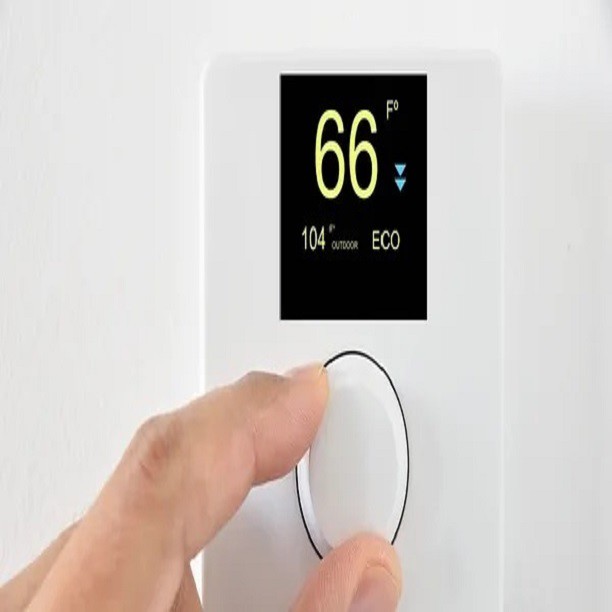In this detailed photograph, a modern smart thermostat is prominently featured, mounted on a pristine white wall. The thermostat unit is entirely white, creating a sleek and minimalist aesthetic. The upper portion of the device is dominated by a tall, black rectangular screen that vividly displays the current temperature in bright yellow digits: 66°F. 

Beneath the screen lies an elliptical white button, which is central to the thermostat's control functions. A human hand is seen interacting with this button; only the index finger, part of the thumb, and a portion of the middle finger are visible, suggesting an adjustment is being made. Two small blue arrows adjacent to the temperature reading indicate that the setting is being changed to a lower temperature.

Additionally, the thermostat's digital display includes a line of white text below the temperature reading. This text states "104 Outdoor ECO," suggesting it provides additional information such as the outdoor temperature and possibly an eco-friendly mode.

The overall design and functionality hint that this is a contemporary smart thermostat, designed for both ease of use and energy efficiency.